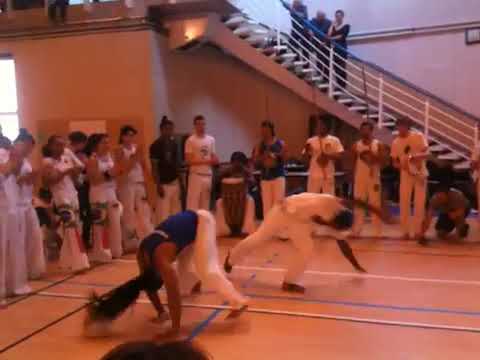This indoor photograph captures a dynamic scene likely depicting a capoeira event, a Brazilian martial art that combines elements of dance, acrobatics, and music. The image is set in a spacious event area with wooden floors and beige walls. At the upper right corner of the background, a long and tall staircase filled with spectators can be seen, with some onlookers standing near the top.

At the center of the image, the focal point, are two individuals in motion. On the left, there is a woman dressed in white pants and a black tank top. She is bent at a 45-degree angle at the waist, with her knees also bent, and her arms are extended with her hands flat against the floor. Her long black ponytail arcs downward as she moves. To her right, a man dressed in white pants and a white short-sleeved shirt mirrors her posture. He, too, is bent at the waist with his knees bent, his right leg slightly lifted off the floor behind him, and his left hand supporting him on the ground. Both individuals appear to be engaged in a sequence of capoeira movements, their heads downward and bodies in fluid motion.

Surrounding the pair, a circle of spectators, some dressed similarly in white pants and shirts or dark tank tops, cheer and clap enthusiastically. Some of these onlookers are also participating in the traditional capoeira roda, contributing to the rhythmic music essential to the practice. The presence of instruments such as conga drums and a berimbau, held by some of the participants, accompanies the performers. This combination of movement, music, and audience participation encapsulates the rich cultural essence of capoeira.